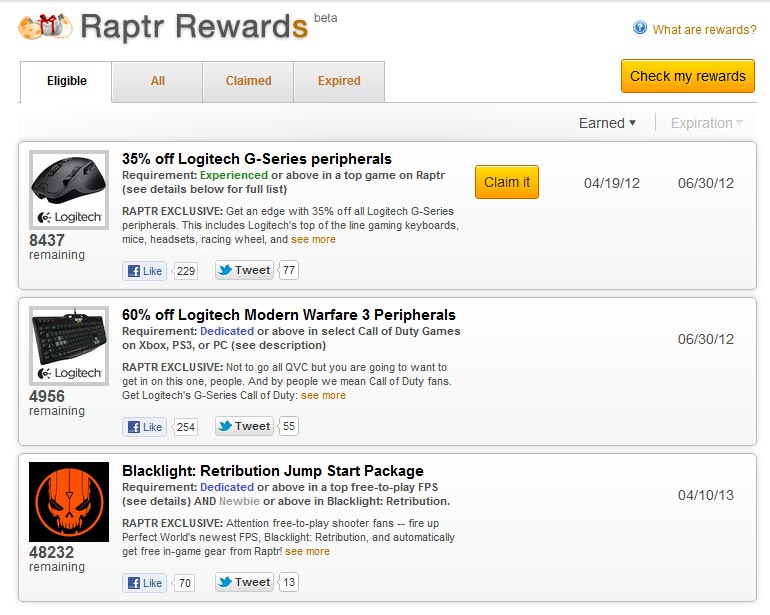The image depicts the interface of the beta version of the Raptor Rewards desktop application. 'Raptor' is distinctly marked on the top left corner, indicating the name of the application. To its right, there is a clickable circular blue logo labeled 'What are rewards?', which likely provides additional information about the reward system. Directly below, a prominent yellow button labeled 'Check my rewards' is displayed, guiding users to check their accumulated rewards.

On the left, there is a tab section with the word 'eligible' highlighted, indicating that this tab is currently selected. Adjacent to 'eligible' are tabs labeled 'all' and 'claimed and expired', offering different views of the user’s rewards status.

Under the 'eligible' tab, the first reward listed provides a 35% discount on Logitech G Series peripherals, with 8,437 of these discounts remaining. The requirements for this reward specify that users must be 'experienced or above' in a top game on Raptor, with further details accessible below. This offer is marked as a 'Raptor exclusive,' highlighting it as a special deal. The discount applies to various top-of-the-line Logitech gaming products, including keyboards, mice, headsets, and racing wheels. The offer has garnered 229 likes and 77 tweets, indicating its popularity. To the right, a yellow button labeled 'claim it' stands ready for users to redeem the reward. Above this button, there's a dropdown menu labeled 'earned,' suggesting it contains previously earned rewards. The date '04/19/12' specifies when the reward was added, and it expires on '06/30/12'.

Below this offer, another reward offering a 60% discount on Logitech Modern Warfare 3 peripherals is listed, with the same expiration date of '06/30/12'. Further down, there is a reward for a 'Blacklight Retribution Jumpstart Package' with an expiration date of '04/10/13'.